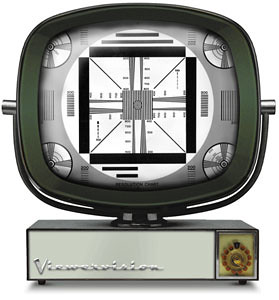The image depicts an antique TV or monitor with a square screen featuring rounded edges and encased in a dark green frame. The interior of the screen showcases a gray chart with distinctive circular patterns at the corners. Each circle has centers composed of a blend of white and gray, and a prominent white circle sits at the center. Within this white circle, there are black squares positioned at the top, bottom, left, and right, just barely touching. Gray lines extend from each corner to a central meeting point, where a smaller gray circle is located. The screen also has thin lines intersecting through it, creating a somewhat propeller-like appearance.

Beneath the screen, there's an attached control box with a light green front panel. Chrome letters are affixed to the front, although they are not legible. The control box, which is long and horizontal, has a noticeable gold-colored knob on the right side, adorned with small red dots around its edge. The object combines vintage aesthetic with functional elements, suggesting it could be a significant piece either for a home or a professional setting.